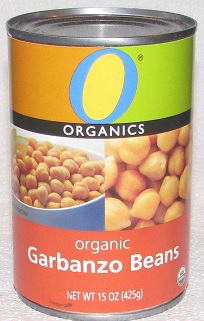This detailed photograph of a silver can of garbanzo beans, set against a gray background, resembles an online product image that allows for an expanded view of the item. The can stands upright with the lid still attached and features a colorful label that encircles the can. At the top of the label, a blue letter "O" is prominently displayed, filled with a gradient of yellow on the left and green on the right. Below the "O," a black strip contains the word "organic" in white letters. Central to the can are two images showcasing the garbanzo beans: the left image displays them in a light blue bowl, while the right image offers a close-up view of the beans, which are light tan and circular in shape. Segregating these images from the lower part of the label is a dark orange band with white text that reads "organic garbanzo beans, net weight 15 ounces, 425 grams." Just beneath the label, a sliver of the metal lip of the can is visible at the bottom.